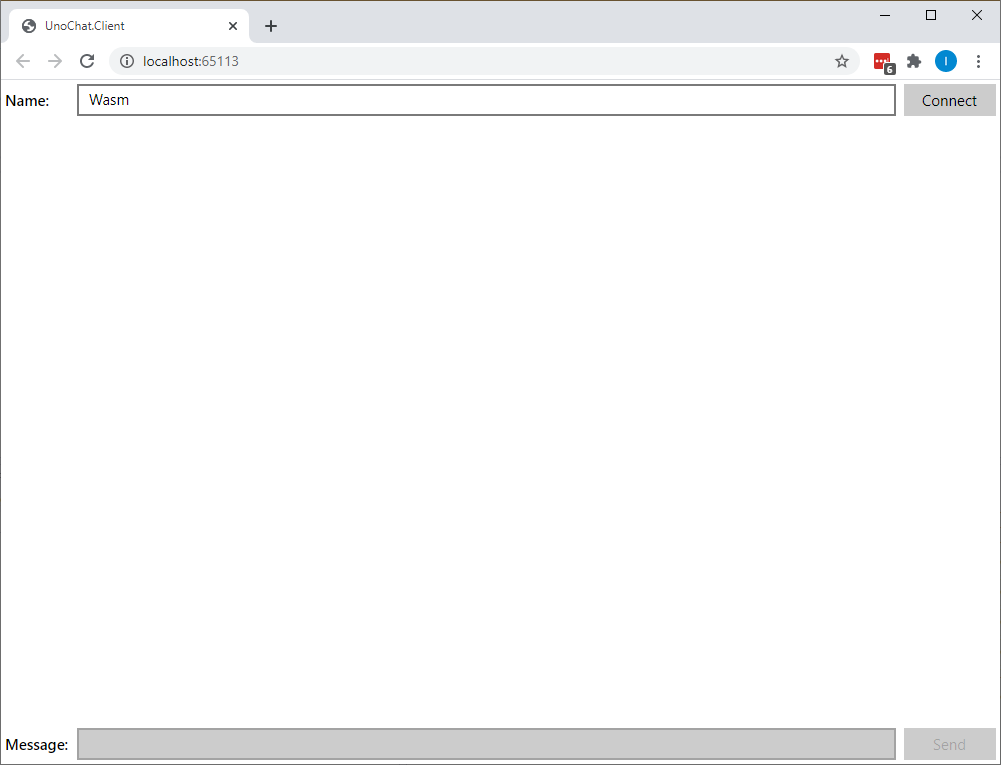The image is a screenshot displaying a computer interface, primarily featuring white and gray tones. Dominating the top left corner is an icon of a planet in gray, accompanied by the text "uno.chat.client." Below that, the address "localhost:65113" is listed. Beneath this, there is a label "Name" adjacent to a lengthy input field, currently reading "wasm" (spelled W-A-S-M). Toward the upper right corner, a gray rectangular button labeled "Connect" is visible.

The rest of the interface is starkly white, with minimal elements until reaching the bottom. Here, on the bottom left, the word "Message" is prominently displayed in black, followed by a sizable gray input box intended for typing messages, which is currently empty. Positioned in the bottom right corner, another button labeled "Send" can be found, which appears to become active once a message is typed in the adjacent input box.